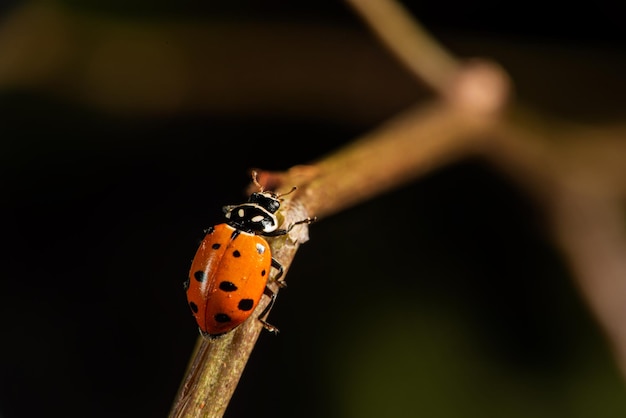This professional, close-up photograph captures a vivid ladybug clinging to a stem as the primary focal point. Dominating the forefront of the image, the ladybug's intricate details are in sharp focus, contrasting sharply with the blurred, out-of-focus background. The stem, curving upward and to the top left corner, creates a natural path that enhances the ladybug's prominence.

The ladybug itself features a striking combination of colors and patterns: a black head and an oval thorax adorned with four white dots, transitioning to an orange-red abdomen. The abdomen is shielded by a hard shell split down the middle, displaying a pattern of black spots—five on one wing and four on the other. The insect’s black legs grip the stem securely, while its antennae extend forward. The backdrop, a blend of light and dark green hues, further accentuates the vivid detailing of the ladybug and stem, adding a sense of depth and natural context to the composition.